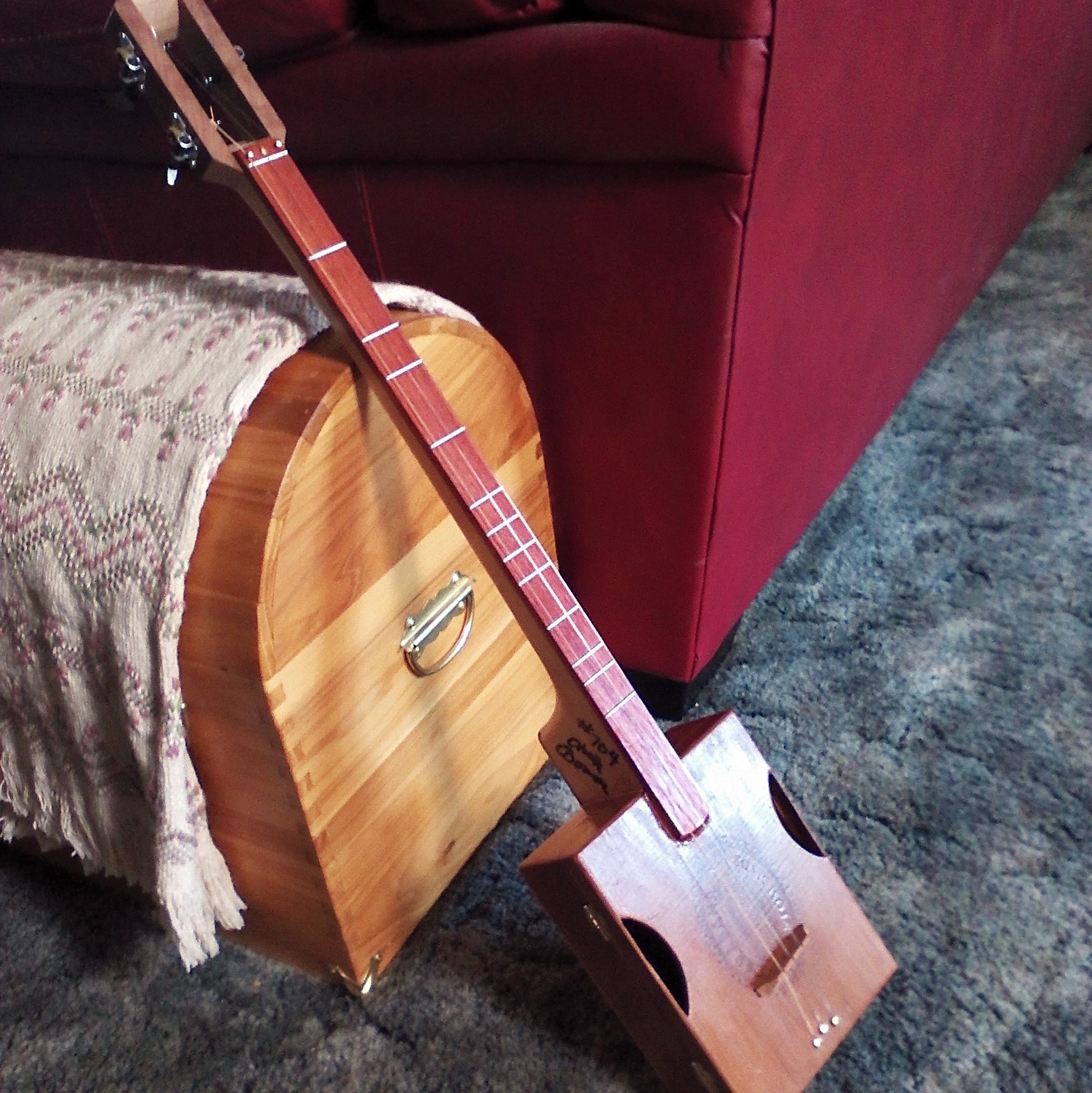In this photograph, there is an unusual, homemade guitar with a distinctive square body, resembling a cigar box, and a small strumming area. The guitar has a reddish walnut-colored fretboard with four tuning pegs, indicating it has four strings. It leans diagonally against an old wooden chest, which is draped with an antique-looking white blanket showcasing pink and dark green designs. The chest, reminiscent of a pirate's treasure chest, is made out of wood, possibly cedar. Behind it sits a maroon or very dark pink couch, similar in color to the guitar's fretboard. The scene is set on a gray shag carpet, possibly in a living room.